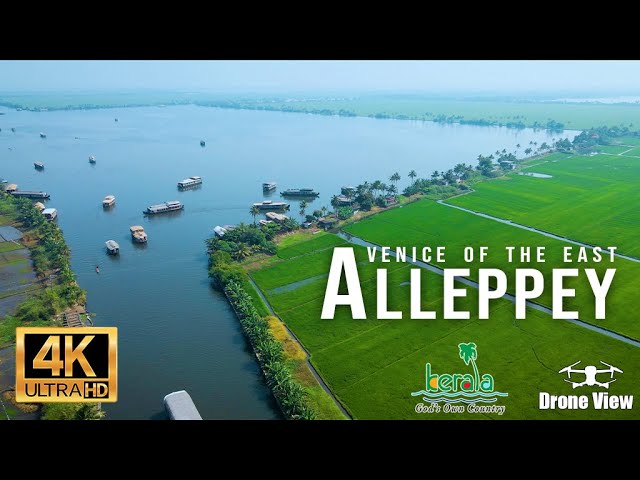The image is a detailed aerial view captured by a drone, showcasing a serene, square-shaped, light blue body of water filled with numerous boats. This water body is situated towards the left side of the image and transitions into a larger canal extending from the bottom left corner. The canal is flanked by tall, lush green trees. On the right side, expansive farmland with rich, green fields appears, intersected by smaller canals. The background is slightly hazy, but additional farmland is visible in the distance. The vibrant green landscape remains mostly undeveloped and free of any residential structures.

In the bottom left corner of the photograph, a gold and black rectangular logo reading “4K Ultra HD” is prominently displayed. To the right, within the green land, white text spells out “Venice of the East Aleppey    A-L-L-E-P-P-E-Y.” At the very bottom right, there's an illustration of a white drone with the label “Drone View.” Nearby is another logo that features the word “Kerala” with a pine tree incorporated into the design, underscoring the region’s identity as “God's Own Country.”